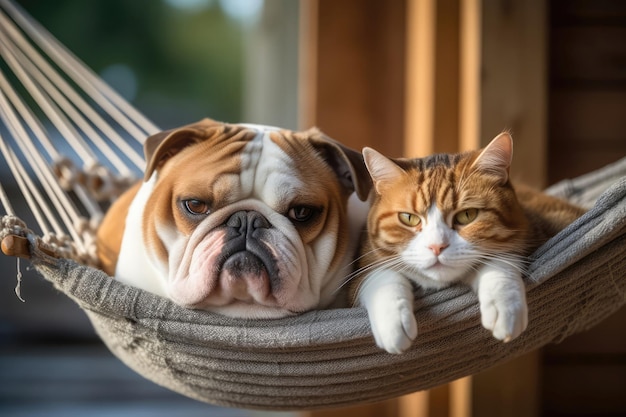In this charming and heartwarming photograph, a light brown and beige English Bulldog with white spots and brown eyes nestles comfortably beside a small orange and white cat in a grey hammock. The bulldog, identifiable by its squishy face and short, floppy ears, exudes a calm and stoic presence. Meanwhile, the cat, with golden-green eyes and a mischievous expression, has its white paws draped casually over the side of the hammock, adding a sense of relaxed whimsy to the scene. The cat's light pink nose and white mouth contrast with its orange and brown fur, creating an endearing visual harmony with its canine companion. Set against a backdrop of a wooden wall with a see-through window revealing greenery, the image captures a serene moment of companionship and tranquility. The hammock, made of plain cloth, seems tailored by circumstance rather than design, perfectly cradling this unlikely duo in what is undoubtedly a picture-perfect moment.